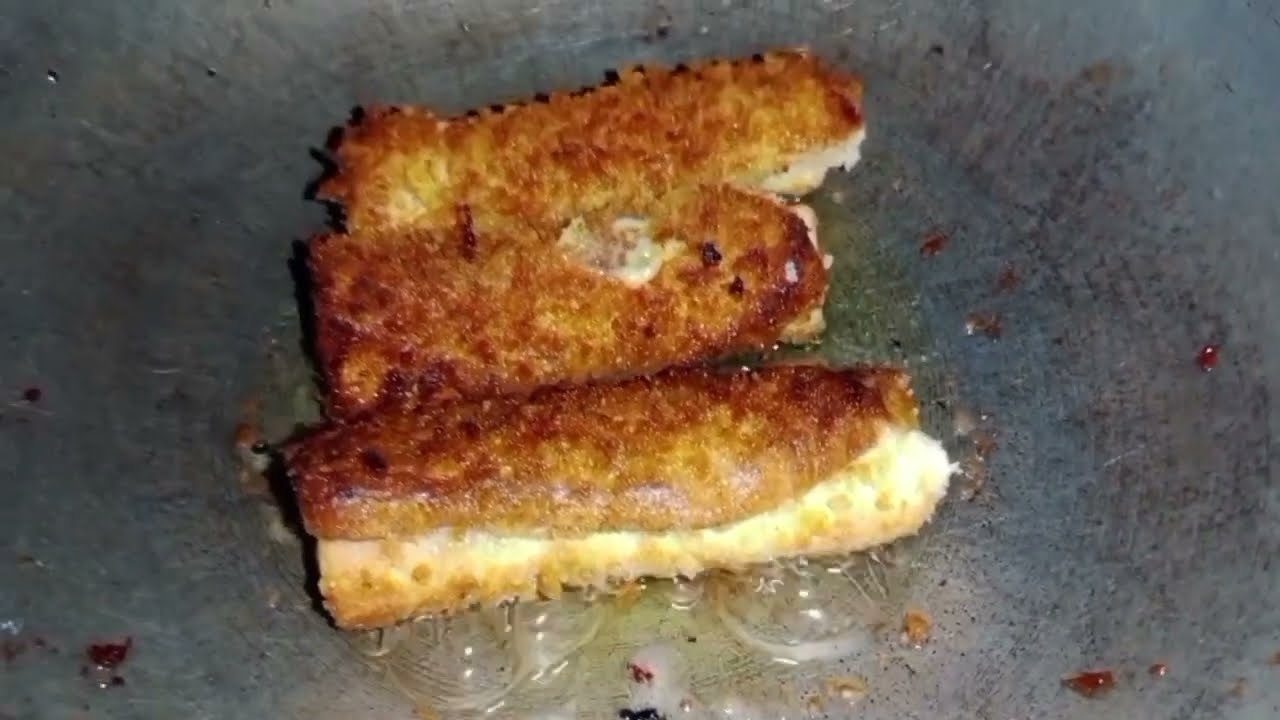The image depicts a close-up view of three food items frying in a silver-colored pan with a slight slope and a flat disk center. The pan has faint rings towards its center and a few burnt spots likely originating from the food. The food items are long and rectangular with curved ends, uniformly brown on top with a coating, and white underneath. Although there's some ambiguity, the items resemble fried bananas or perhaps fish sticks, though they're slightly different in shape and style, with one having more coating than the others. The food is arranged horizontally relative to the camera, which looks down on them. Visible bubbles of oil, especially around the item in the front, suggest the frying process is ongoing. The background is a grayish surface, adding a stark contrast to the golden-brown, crisped texture of the food, enhancing its visual appeal.